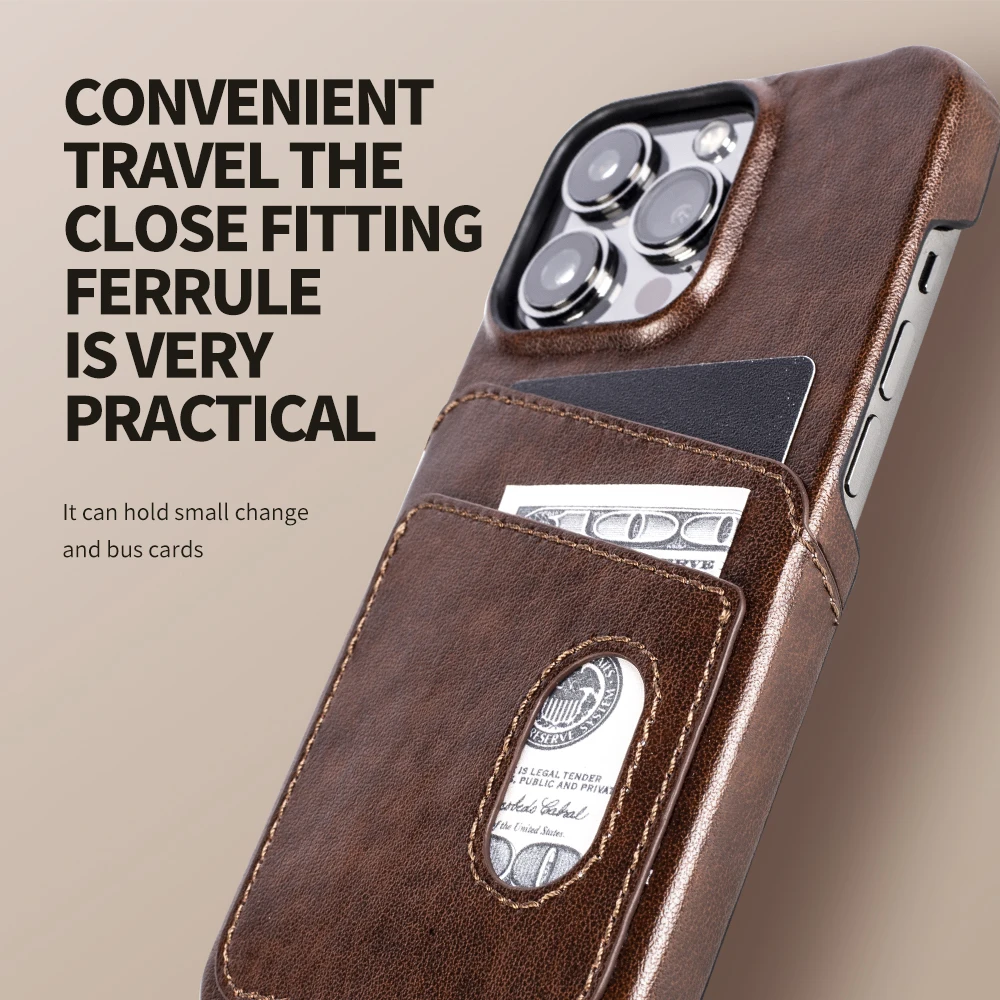This advertisement features a detailed image of a brown leather phone case designed for iPhones, doubling as a wallet. The phone case prominently displays two back pockets: the top pocket holds a black card, while a $100 bill peeks out from the bottom pocket, which features a small hole, likely for easy access to an ID. The case has precise cutouts for a three-lens camera and side buttons. The background of the image is a light brown or puce color, complementing the case. On the left side of the image, bold black text reads, "Convenient travel. The close-fitting Ferrule is very practical." Beneath it, smaller text explains that the case "can hold small change and bus cards."